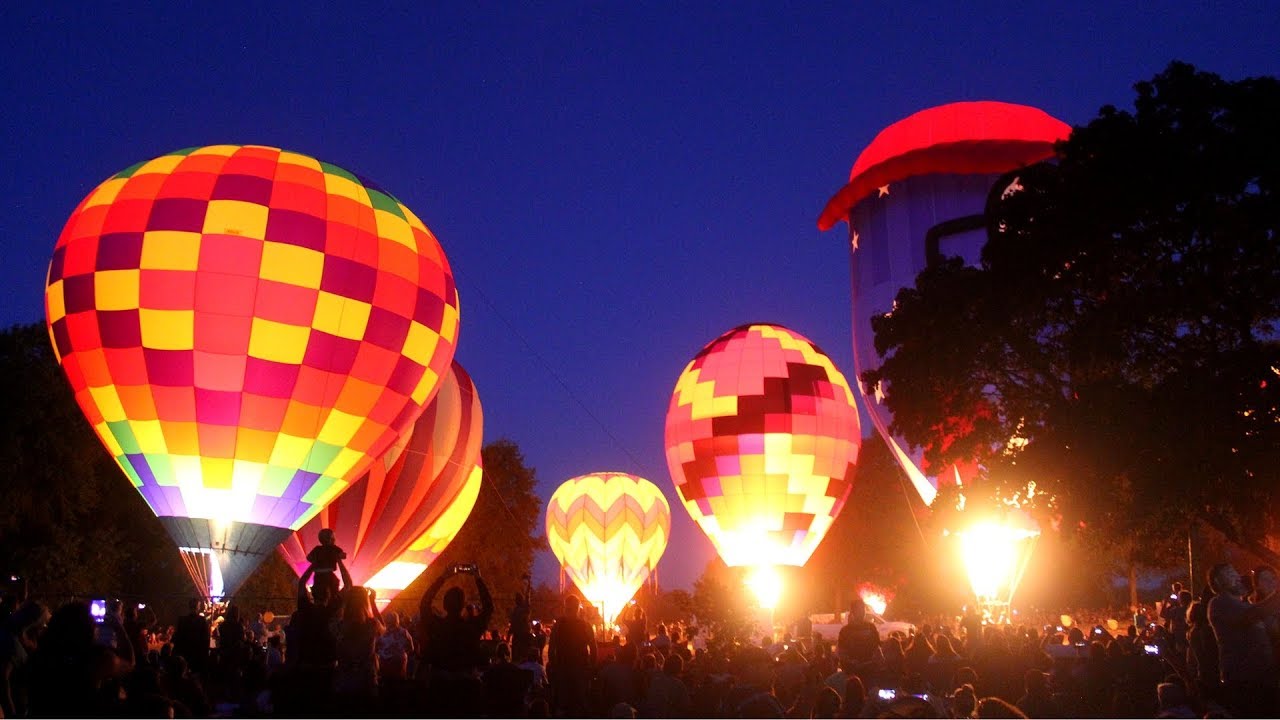This color photograph captures a vibrant nighttime scene at a hot air balloon festival. The dark indigo sky forms a stark contrast against six brightly lit hot air balloons, each adorned with vivid, multicolored patterns, including a mosaic of red, orange, yellow, and green squares, and chevron designs. The flame-heated balloons illuminate the surrounding area, casting light on a large crowd. Some people are seen holding up cell phones, capturing the mesmerizing view, and one man is lifting a child onto his shoulders, the child gazing in awe at the balloons. In the background, there is a peculiar structure with a red roof, which could be a water tower or a creative element, and a large silhouetted tree stands to the right of the image. A truck is also visible behind the crowd, possibly on standby for safety.